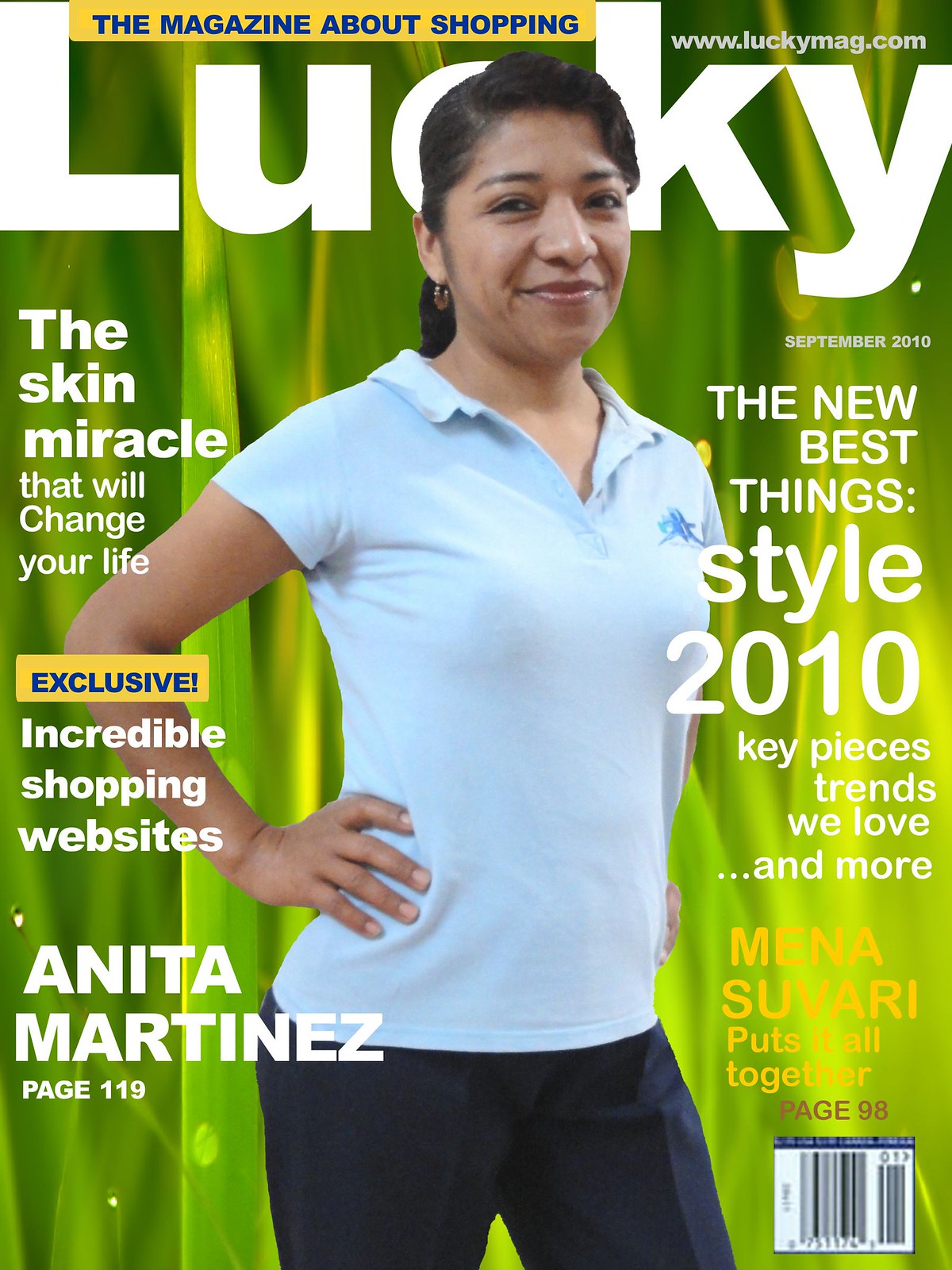The magazine cover is vertically aligned, featuring the title "Lucky" prominently at the top in large white block letters, although the "C" is partially obscured by the central figure. The tagline "the magazine about shopping" appears in smaller, all caps blue letters alongside the magazine's website, www.luckymag.com. The background is predominantly green with textured leaves visible, providing a vibrant contrast to the other elements on the cover.

At the center of the cover is a woman named Anita Martinez, identified by bold, all caps white letters on the lower left-hand side, along with a reference to page 119. She is smiling warmly, her dark hair and eyes complementing her outfit: a light blue, short-sleeved polo shirt with a logo on the left chest, paired with dark blue pants. Her hands rest on her hips, and only her upper body is visible.

Highlighted article titles are scattered across the cover. On the left side, in bolded white letters atop one another, is the phrase "The Skin Miracle That Will Change Your Life." Directly beneath, a small yellow rectangle with all caps blue letters reads "Exclusive," followed by "Incredible Shopping Websites" in white font. Over on the right side, the text "The New Best Things" is right-aligned in white. Below that, it states "Style 2010, Key Pieces, Trends We Love and More." Further down, in yellow letters, it says "Mina Suvari Puts It All Together," with a reference to page 98 underneath.

This issue is from September 2010, as indicated on the right side of the cover, and a barcode is positioned at the lower right-hand corner.